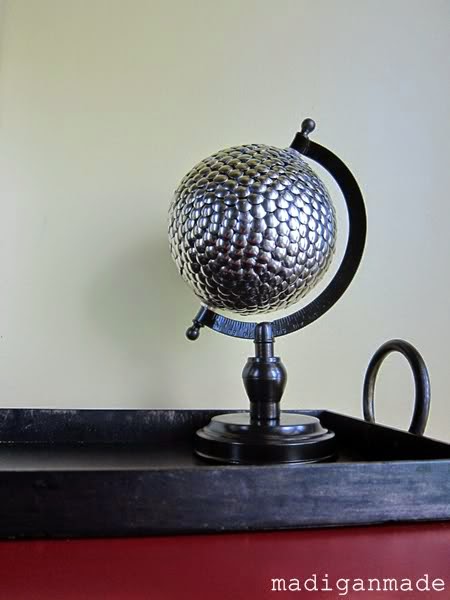In this image, a unique globe is showcased, distinguished not by the usual geographical depiction, but by its surface of hammered, silver metal scales resembling those of a lizard or fish, forming a mix of square and hexagonal patterns. The globe, approximately four to five inches in diameter, is cradled by a black or oil-rubbed bronze pedestal, typically found supporting traditional globes. This assembly is perched on a black tray which features a large ring handle on its right side. The tray rests on a red or maroon table, within a room characterized by white walls and a neutral-toned background that casts a shadow of the globe. In the bottom right corner, the image is subtly marked with the copyright name "Madigan Made," spelled out as M-A-D-I-G-A-N M-A-D-E. This minimalist, yet striking setup highlights the artistic blend of metal craftsmanship and everyday objects.